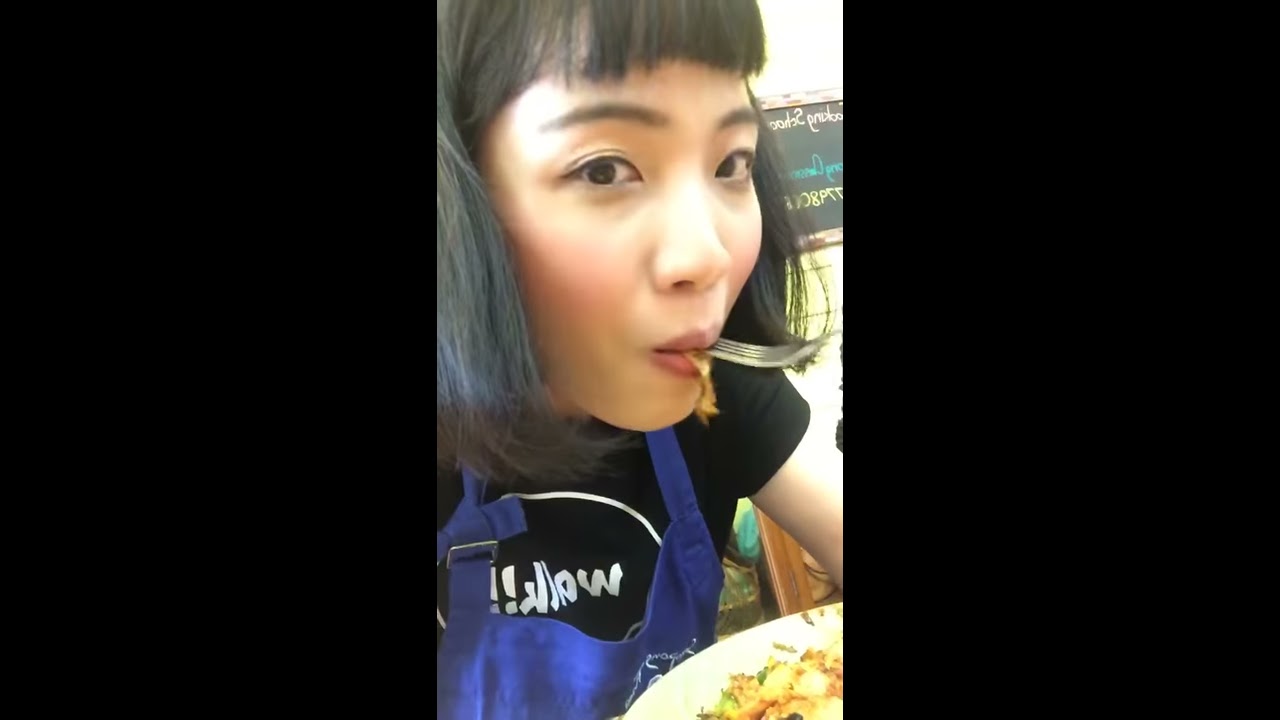The image depicts a young Asian woman with long black hair and soft brown eyebrows, her face positioned centrally with black borders on either side. She is dressed in a black shirt featuring backwards white text that includes "K," "L," an "E," and a "W," as well as two exclamation marks. Over her shirt, she wears a blue apron adorned with a white design. The woman has pink lips, rosy cheeks with pink blush, and brown eyes. She appears to be eating, as a fork extends from the right side of the image into her mouth, with a piece of tan-brown food dangling from her lips down to her chin. In front of her, in the lower right corner, is a white plate holding brown food and what looks like green peppers or peas. The setting suggests an indoor environment, complemented by a visible brown chair and a slightly obscured blackboard with writing behind her. The focal point is her face, framed with long bangs and curving hair, alongside the fork in her mouth.